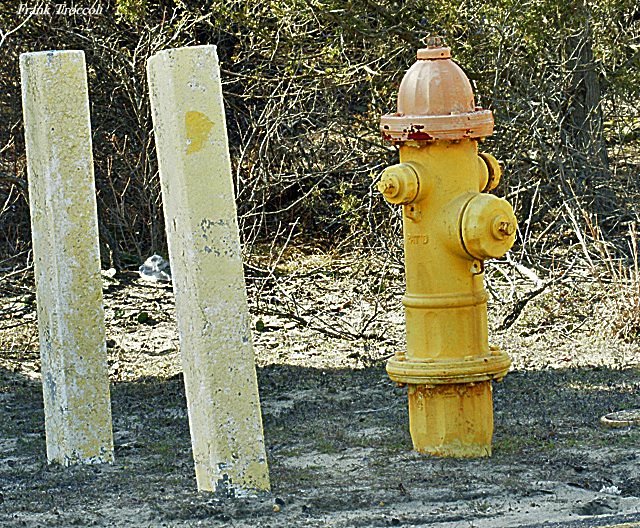This photograph captures a scene featuring a prominent yellow fire hydrant with a faded brownish cap situated in a dirt-filled, cracked pavement area. To the left of the fire hydrant, two pale yellow, weathered concrete posts are embedded in the ground, appearing to have once been painted but now show signs of wear and cracks. The ground is old and cracked, with small patches of grass emerging from it, interspersed with gravel, rocks, and debris. In the background, there is a dense array of trees and foliage, displaying a mix of green leaves and brown tree trunks and branches, suggesting a somewhat neglected and overgrown area. The environment looks sunlit, though the fire hydrant and posts are in the shade, while sunlight highlights the vegetation in the background.